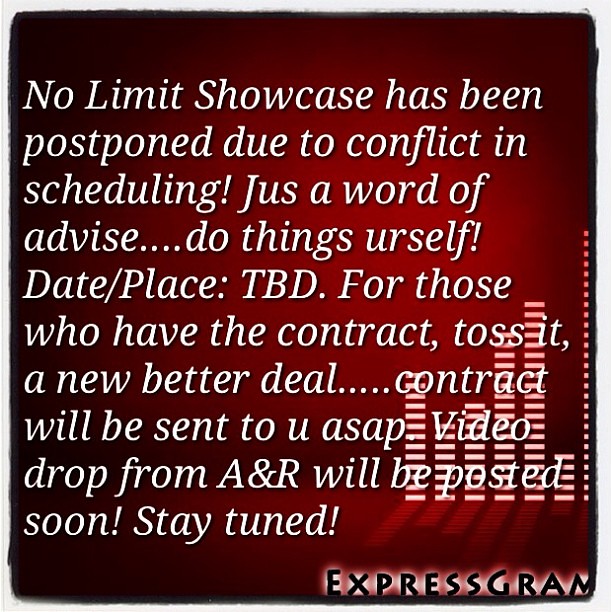The image features a digital announcement with a stark red background and white text. There is a vignette effect, creating a dark-to-light gradient from the corners to the center. Overlaid on the background are bar-like sound equalizer visuals and white dots in the bottom right corner. The message reads: "No Limit Showcase has been postponed due to a scheduling conflict. Just a word of advice: do things yourself. Date and place to be determined. For those with a contract, toss it. A new, better deal contract will be sent to you as soon as possible. A video drop from A&R will be posted soon. Stay tuned." At the bottom, "Expressgram" is displayed in distinctive black text with a glowing white frame around it.